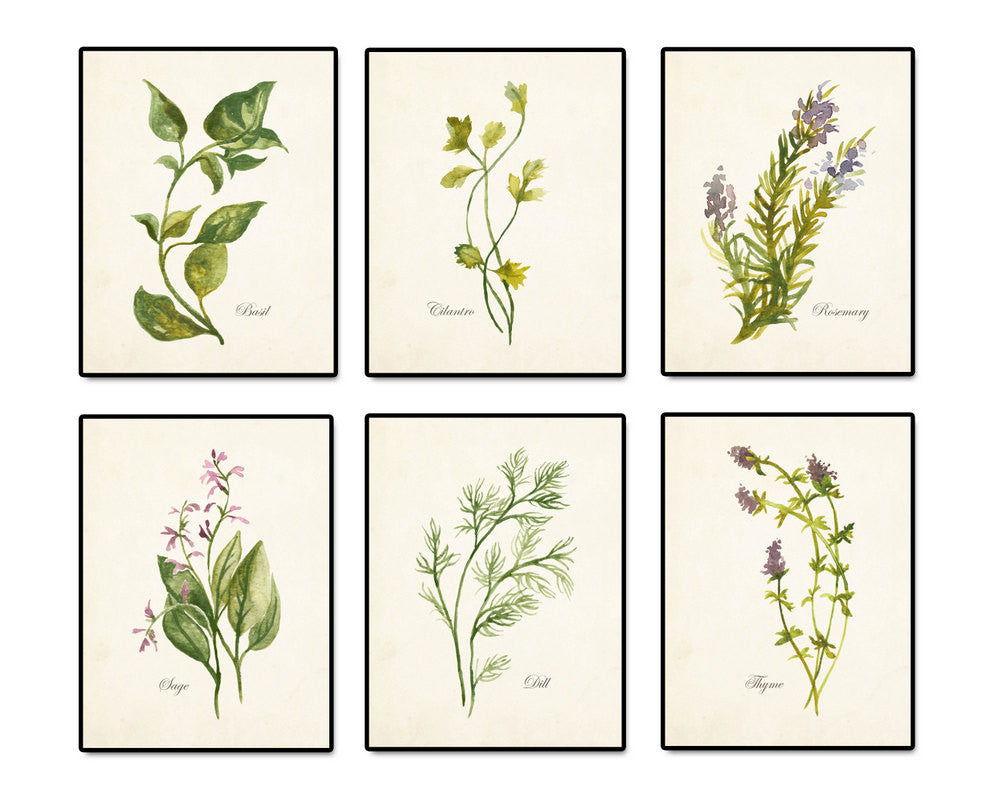The image showcases a collection of six framed botanical artworks, each meticulously arranged on a white wall and featuring black frames with tan matting. Starting from the upper left, the first artwork displays a vibrant green basil plant, characterized by a central stem and outward-arching leaves, labeled "basil" at the lower right corner. Adjacent to it in the center is an illustration of cilantro, with its distinctive upward-pointed stems and delicate, feathery leaves. The upper right artwork portrays rosemary, notable for its needle-like green leaves and a pale lavender flower at the tip.

On the lower left, there's an artwork depicting sage, detailed with textured green leaves and small pink flowers. The center lower frame features dill, recognizable by its wispy, delicate leaves resembling fine needles. Finally, the lower right artwork illustrates thyme, with green stems adorned by tiny leaves and small clusters of purple flowers. Each piece elegantly captures the unique characteristics of the plants, creating a harmonious display of botanical beauty.